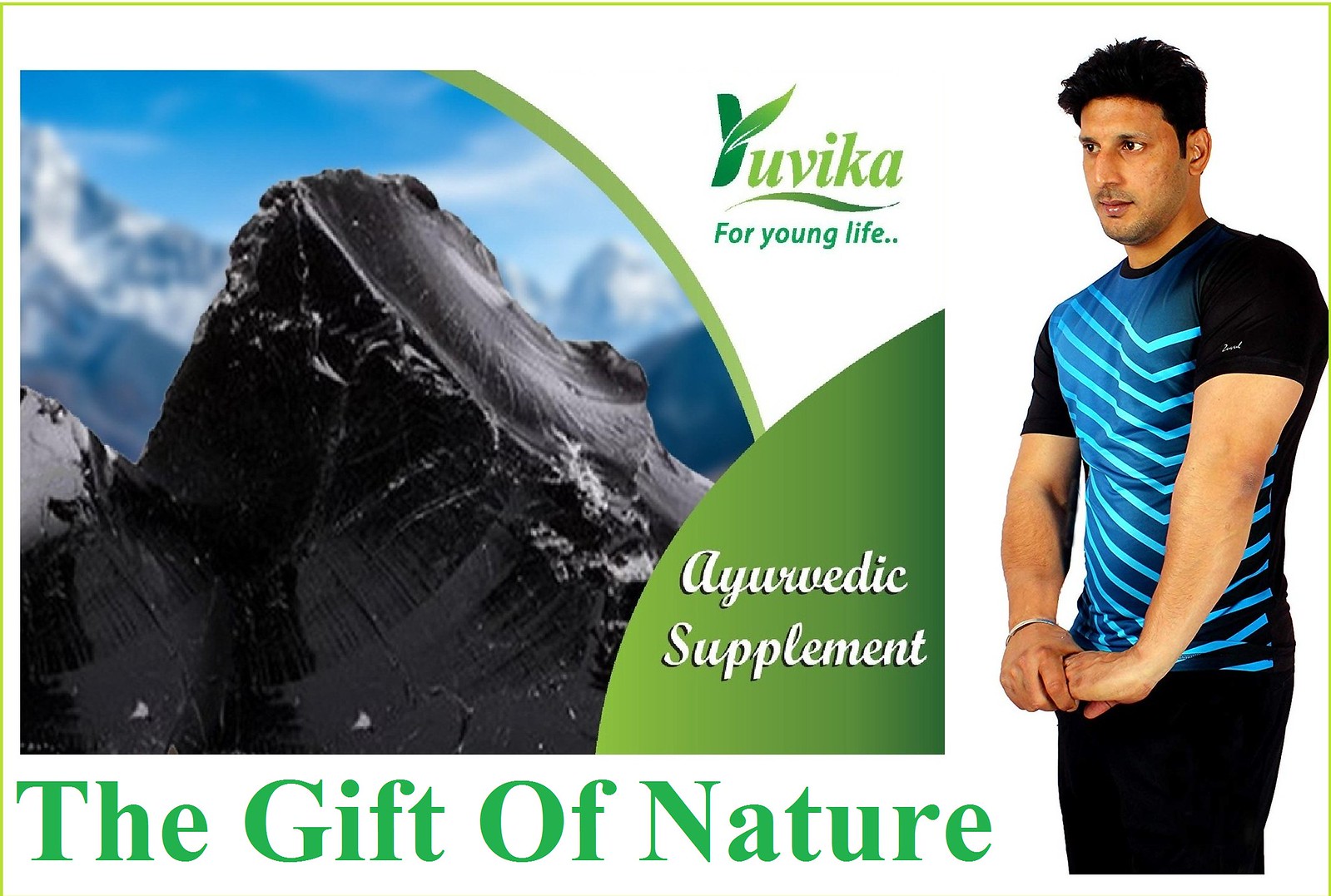This advertisement photograph for an Ayurvedic supplement, titled *UVICA for Young Life*, showcases a scenic background featuring a mountain with a blue sky and white clouds, surrounded by a green semicircle. The prominent logo "UVICA for Young Life," rendered in green with a leaf graphic on the capital "Y," is displayed at the top. Below the mountain image, the phrase "the gift of nature" is written in green. To the right, there is a photograph of a young, muscular South Asian man with short black hair and a long nose. He is dressed in black pants and a short-sleeved t-shirt with blue and light blue stripes across the chest. The man appears to be either stretching or examining the image in front of him. At the bottom right, the term "Ayurvedic supplement" is highlighted in white text.